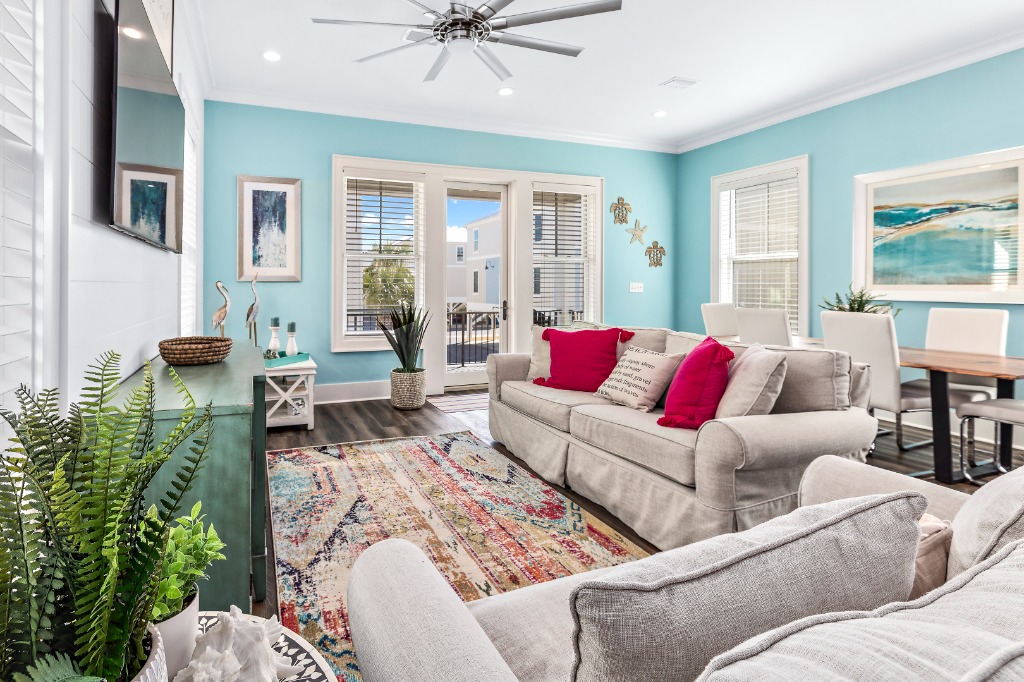The photograph captures a beautifully designed, cottage-style living room brimming with coastal charm. The serene space features soft blue walls and a crisp white ceiling complemented by a silver ceiling fan. Taupe-colored sofas with red and beige pillows provide ample seating, paired with a distressed green console adding a touch of rustic elegance. Nautical and beach-themed decorations, including turtle designs and sea-inspired artwork in blues and greens, adorn the walls. The room is well-furnished with clean lines and a cozy feel, accented by several potted plants scattered around. A dining area in the background seats six with taupe-colored chairs, contributing to the airy and inviting atmosphere. The overall decor is a blend of contemporary style with coastal elements, making it a perfect vacation rental spot. The sky outside is vividly blue, enhancing the natural light flooding the room, although the view seems to be of other apartments rather than a waterfront. The warm wooden floors are complemented by a colorful throw rug, tying the elements of the room together harmoniously. Candlesticks with teal candles, abstract art, cranes, and shells further enhance the seaside ambiance.